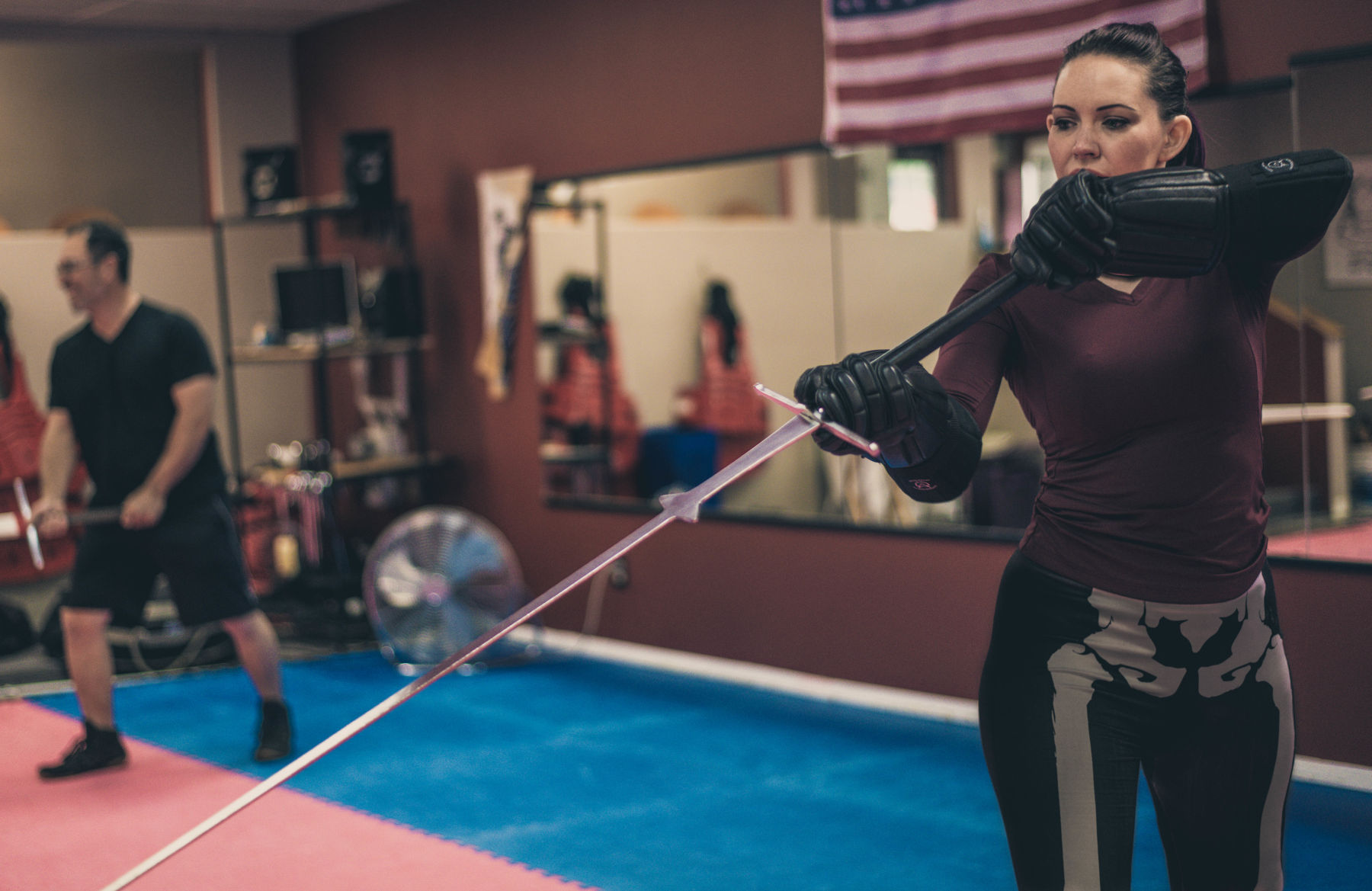In this photograph of a fencing studio, a slightly blurry image captures a woman in sharp focus on the right side. She is dressed in a form-fitting black suit with skeleton bone patterns on the pants. She wears long, black gloves that extend past her elbows and holds a long, thin fencing sword with a black grip and shiny silver hilt, pointing it diagonally downward in front of her as if in deep concentration. Her black hair is pulled back, and her white skin contrasts significantly against her dark attire. 

The background reveals a large mirror reflecting other fencers and a prominently displayed American flag with red and white stripes above it. The studio has a rust-colored wall, and a white bar with a circular clear piece attached runs across it. To the left of the image stands a man in a black t-shirt, dark shorts, black sneakers, and glasses, also holding a sword. He appears happy and relaxed. The floor matting beneath them is bright red with a thick blue border, and other elements in the room include a silver fan on the floor and an open shelf housing black and silver trophies.